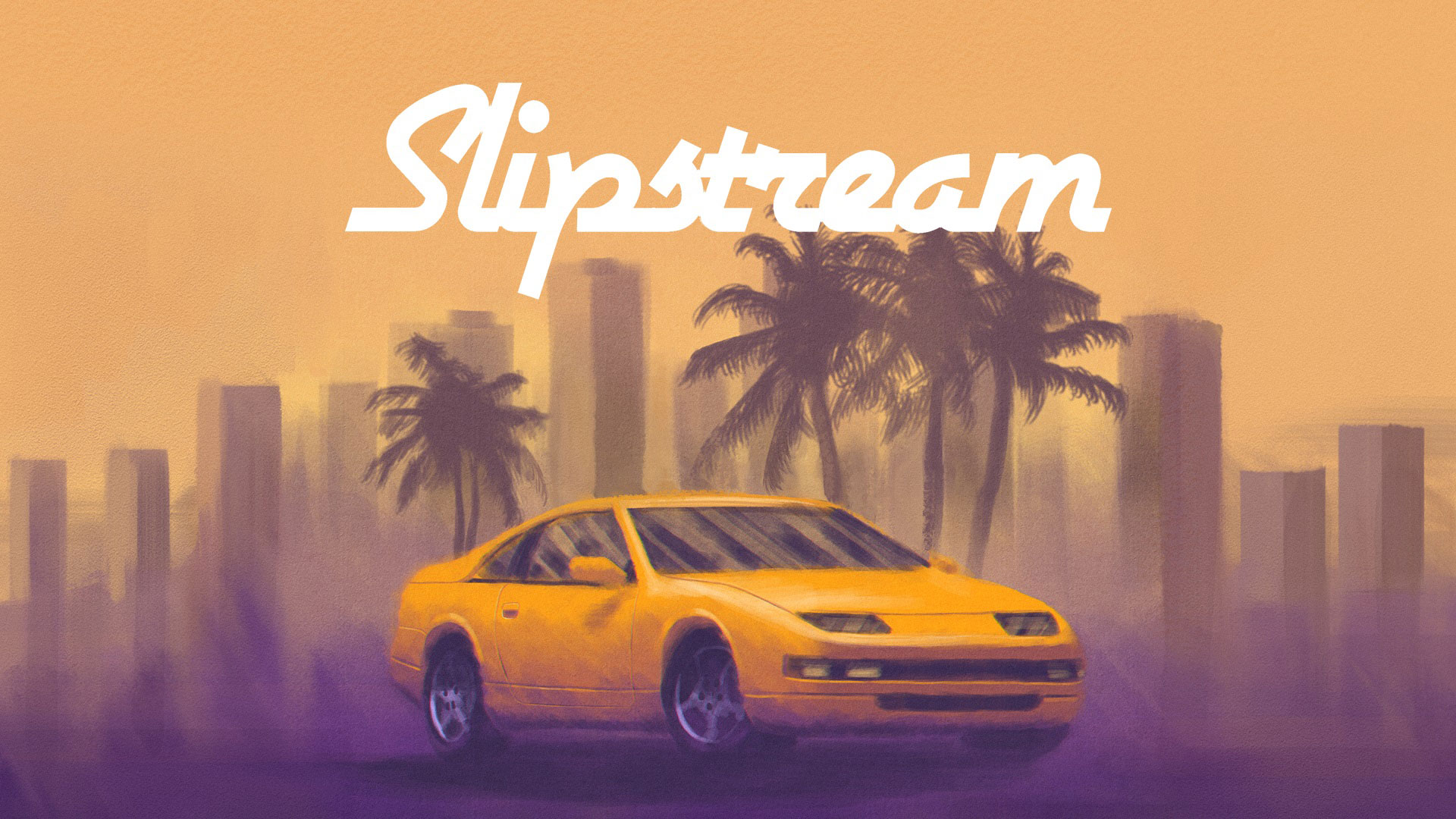This artwork, potentially a computer-generated graphic or a hand-drawn illustration, depicts a vivid scene titled "Slipstream." The background comprises a gradient orange sky, resembling a sunset, which imbues the scene with a warm ambiance. The detailed foreground features a sleek, ornately designed sports car, either in a hue of yellow or orange, with a low-profile front end and nearly concealed lights. The car's right side is prominently displayed, showcasing its polished black tires and silver rims.

Behind the car, there are outlines of skyscrapers rendered in gray, providing a minimalist urban backdrop. The car is flanked by four palm trees: one situated at its rear and three more in front of it. The word "Slipstream," written in white with a capital 'S' followed by cursive lettering, is prominently positioned above the buildings and most of the palm trees, adding a stylish touch to the overall composition. The image's background elements, including the buildings and palm trees, are intentionally blurred, drawing focus to the meticulously crafted car, which stands as the centerpiece of the artwork.